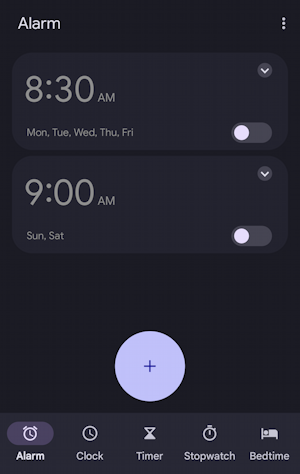This image is a screenshot of the alarm section of a cell phone, characterized by a background in various shades of black. At the top left corner, the word "Alarm" is displayed prominently in white text. In the top right corner, three vertical dots indicate additional settings options. 

The main body of the screen shows two listed alarms. The first alarm is set for 8:30 a.m. and is scheduled to repeat on Monday, Tuesday, Wednesday, Thursday, and Friday. The toggle switch next to this alarm is in the off position, indicating that the alarm is deactivated. Above this toggle switch, a drop-down arrow hints at further customization options.

The second alarm is set for 9:00 a.m. on Saturday and Sunday. Similarly, its toggle switch is also in the off position, with a drop-down arrow above it for more settings.

Near the bottom center of the screen, a light purple circle with a plus sign in the middle provides a quick option to add new alarms.

At the very bottom of the screen, several options related to the alarm function are displayed, accompanied by icons. These options are "Alarm," "Clock," "Timer," "Stopwatch," and "Bedtime." Each option is labeled with an illustrative icon: a small clock above "Alarm," a traditional clock above "Clock," an hourglass above "Timer," a stopwatch above "Stopwatch," and a bed with a person sleeping in it above "Bedtime."